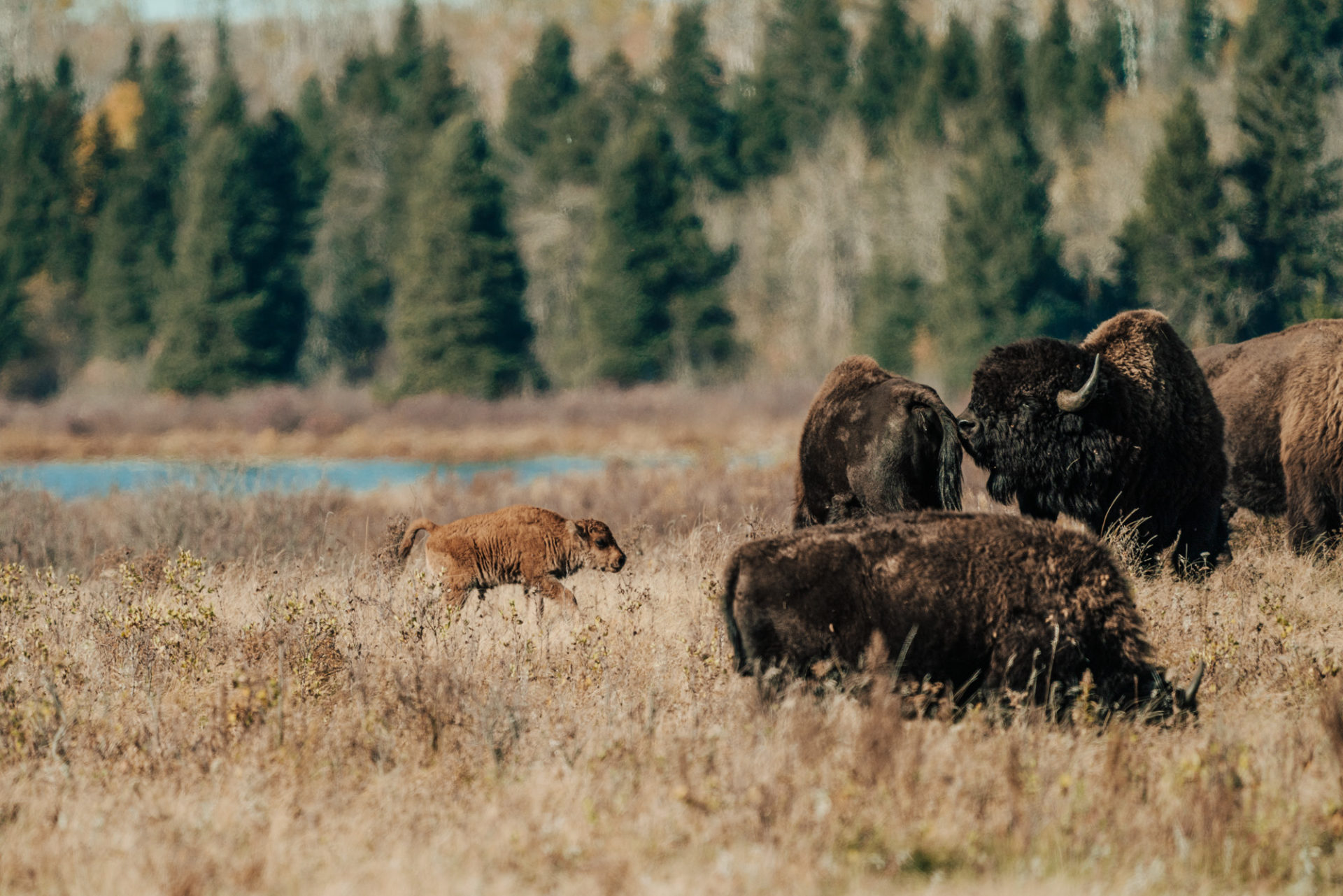The photograph captures a serene, though somewhat desolate, nature scene featuring a partial shot of a herd of buffalo. The setting is a dried-up field with brown, withered plants and grass, indicative of an autumn or winter landscape. In the background, a hill is covered with a mix of evergreen and deciduous trees, some green and others leafless. A single dead tree with golden-yellow leaves stands out among the greenery on the far right. A portion of a crystal blue lake is visible on the left side of the image, adding a splash of color to the otherwise muted tones.

The buffalo dominate the center and right portions of the frame. Three adult buffalo, large with dark black and brown furry bodies and imposing horns, are positioned on the right. One of them bends its head to graze, another's rear is visible, and a third shows its face with a prominent black horn. All appear robust and immense. In the left center, a baby buffalo with wrinkly, light brown fur and an arced tail is captured in motion, galloping toward the adults. The overall composition emphasizes the peaceful yet stark reality of the wilderness, blending the life and death cycles in nature.